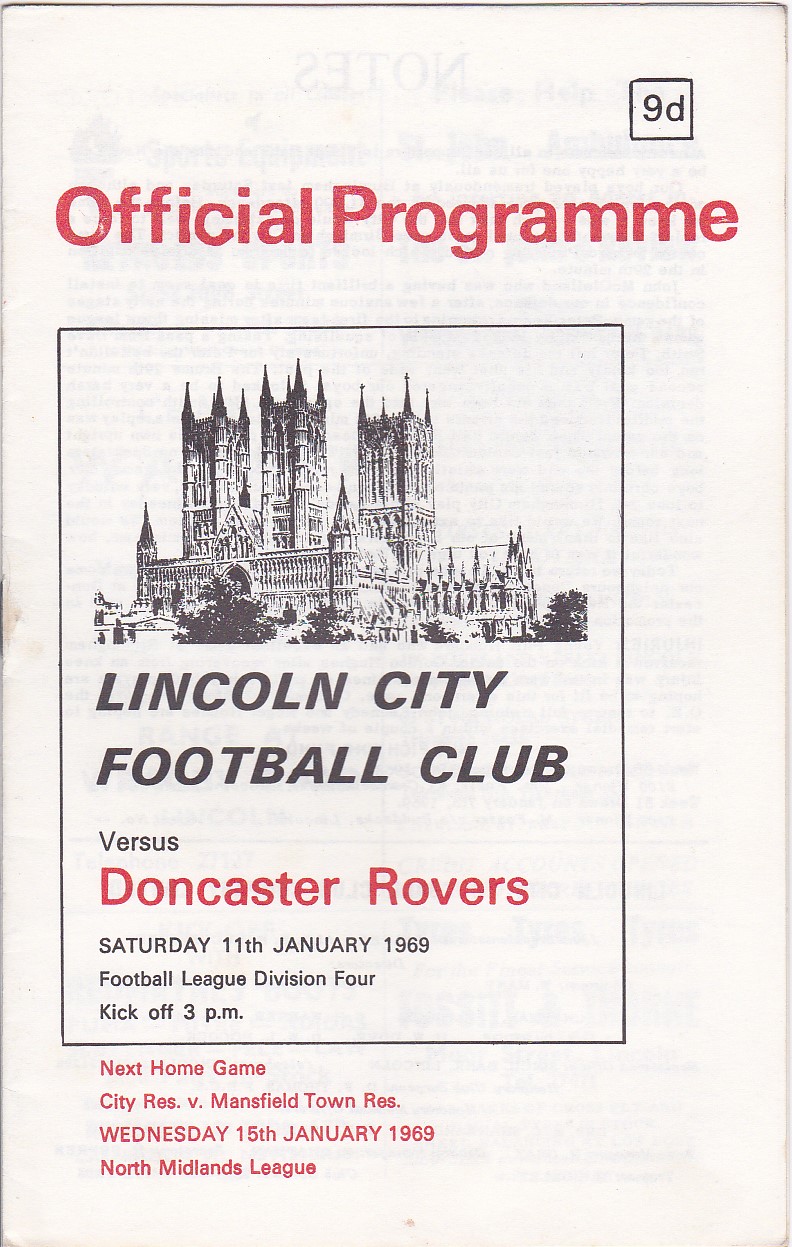The image shows a digital copy of an official football program from the United Kingdom. The pamphlet, formatted on a white sheet of paper, features the title in red text at the top, spelling "Official Programme" in British English. Below this, a small black square with "9D" in black letters, likely indicating the price of nine pence.

Central to the design is another box, predominantly located towards the left side, containing a graphic of a cathedral. Beneath the illustration, in bold, italic capital letters, it reads "LINCOLN CITY FOOTBALL CLUB." The text "VERSUS DONCASTER ROVERS" follows, with "DONCASTER ROVERS" and the team names written in red. Below this, in black text, it states "Saturday, 11th January 1969," indicating the match date, followed by "Football League Division 4" and "Kickoff 3 p.m." in smaller black font. 

The bottom section announces the next home game in red text: "Next Home Game, CITY RES. V. MANSFIELD TOWN RES., Wednesday, 15th January 1969, North Midlands League." The entire layout suggests this is a historical program for the Lincoln City Football Club, detailing their scheduled match against Doncaster Rovers dated January 11th, 1969.